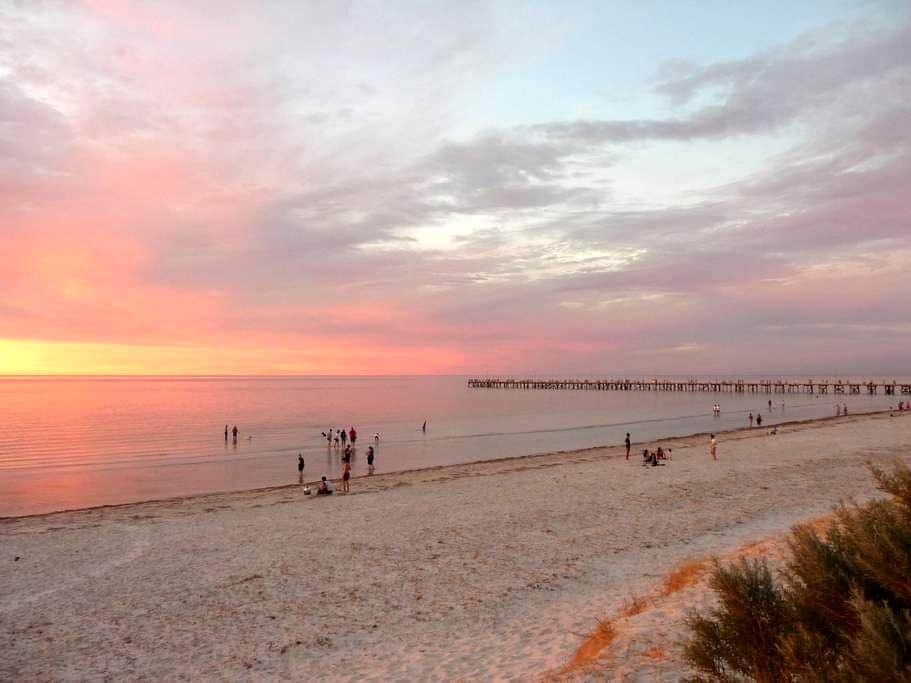This image captures a serene beach scene during what appears to be either sunrise or sunset. The focus is primarily on a tranquil coastal area. In the bottom right corner, a bush can be seen, leading into a sandy beach stretching across the right side of the image, its brown grains illuminated by the warm light. The center of the image showcases calm water, reflecting hues of pink, yellow, and orange from the sky above, indicative of the soft light from the sun just above the horizon. A sturdy brown pier extends from the right-hand side out into the ocean, accompanied by a scattering of people; some wade in the still, reflective water while others mill about the shoreline and the pier itself. The sky covers the upper half of the image, painted in gradients of light blue, gray, and pink, with some clouds drifting through, adding texture to the vast expanse. The atmosphere suggests a warm, inviting, coastal environment ideal for a peaceful retreat.